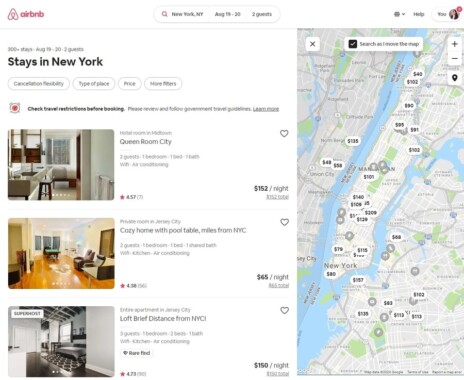Screenshot of an Airbnb listing page showcasing New York City accommodations. The Airbnb logo is prominently displayed in the top left corner. The destination is set to New York City, with selected dates that are difficult to discern due to the blurriness. The search is set for two guests, with the heading "Stays in New York" below. Three primary search results are displayed with accompanying images and descriptions:

1. The first listing features an image of a modern, predominantly white interior. The text to the right, though somewhat blurry, reads "Hotel Room: Queen Room City" and lists the price as $152 per night.
   
2. The second listing shows a cozy living room with wooden flooring, a table, windows in the background, and a chair to the right. The caption reads "Private Room in Jersey City: Cozy home with pool table, miles from NYC," priced at $65 per night.
   
3. The third listing, marked with a "Superhost" badge, displays a black-and-white photograph of a loft. The description reads "Loft: Brief distance from NYC" and is priced at $150 per night.

To the right of these listings, a map of the area is visible with various price labels indicating different accommodations, though the text is blurry and hard to read. The map contains a couple of dozen price markers, providing a visual spread of accommodation costs in the area.